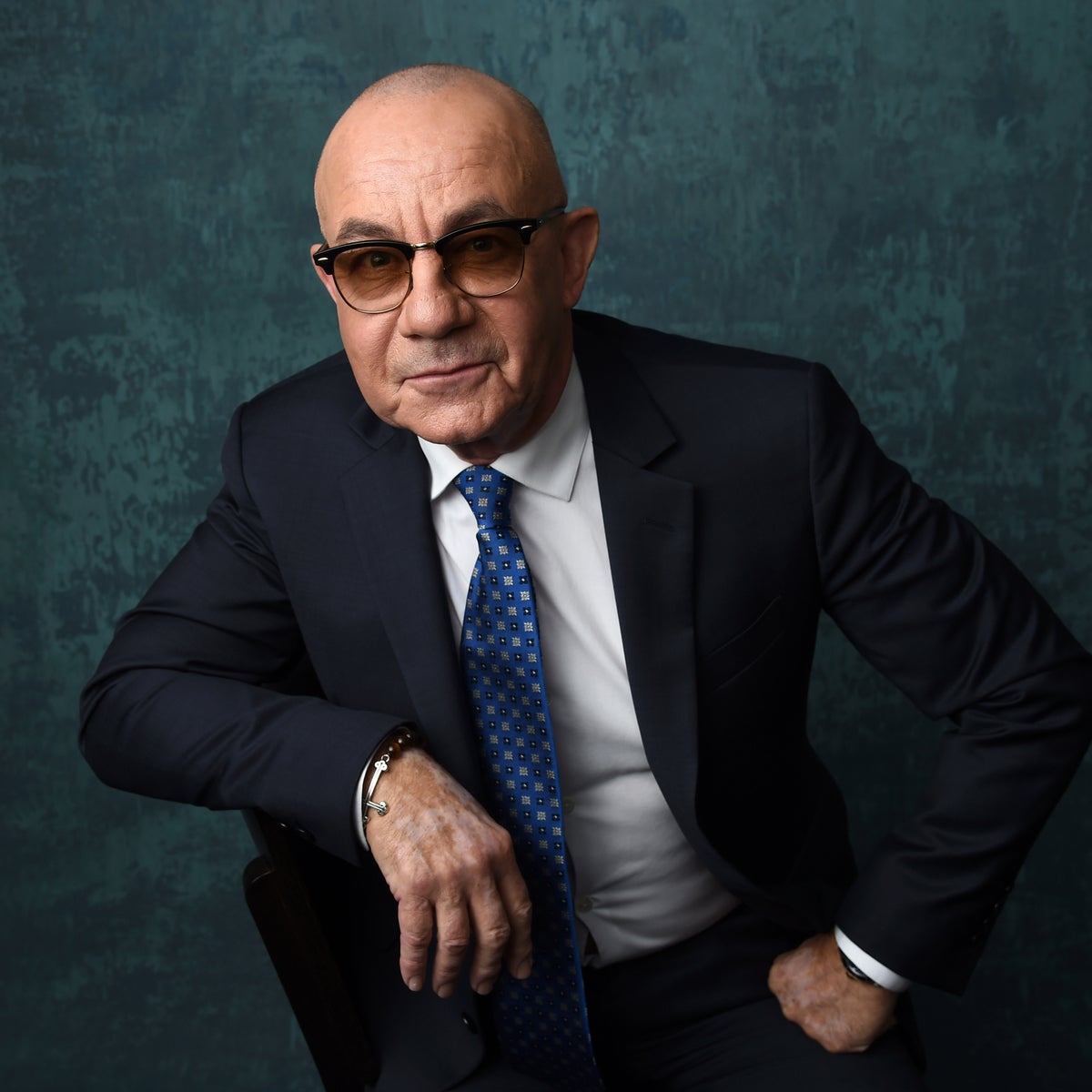This color photograph, presented in a square format, features a detailed portrait of the renowned musical composer Bernie Taupin. The subject, an older bald man with a wrinkled face and liver-spotted hands, exudes a sense of style and sophistication. Dressed impeccably in a dark, nearly black suit with matching pants, Taupin is further refined by a white collared shirt and a blue tie adorned with small square designs. He accessorizes with tinted eyeglasses and bracelets on his right wrist. 

In the portrait, Bernie Taupin is seated in a black chair facing the viewer. His right arm is raised and bent at the elbow, resting on the top of the chair, while his left arm, also bent at the elbow, is propped against his hip. His expression is neutral, with a furrowed brow. The background features a dark teal brush effect, contributing to the photographic realism and representationalism of the portrait. Taupin's polished appearance and poised demeanor suggest a deliberate effort to showcase his enduring sense of style.